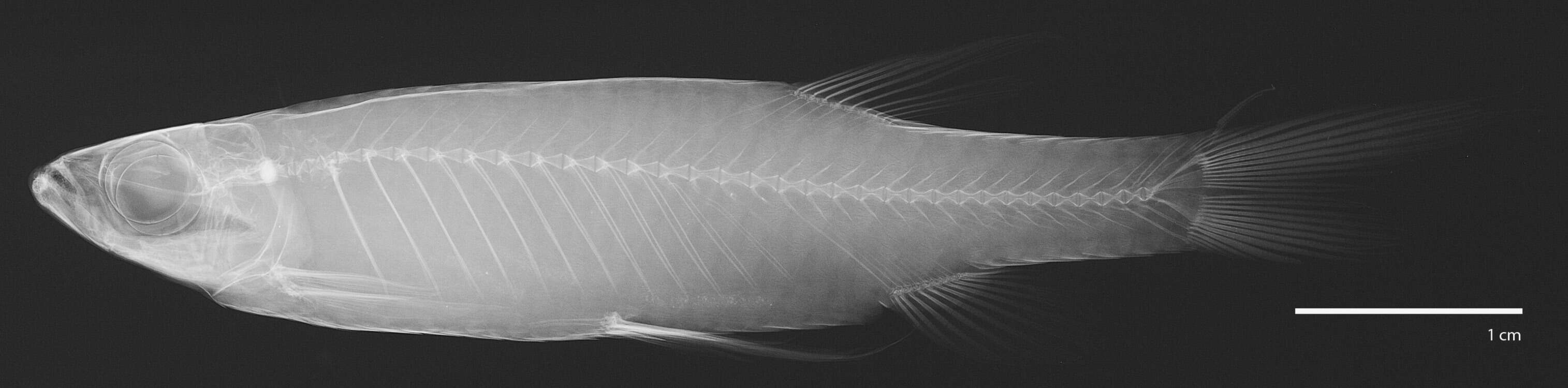This black and white image features an x-ray of a fish, presented in a long horizontal format with a black background. The fish's skeletal structure is clearly visible, with the bones illuminated in a whitish color against the dark backdrop. Positioned horizontally, the fish is facing left, showcasing a detailed side profile. Its large eye dominates much of the head, and its small mouth is also discernible. The spine runs from the head down to the tail, with bones extending diagonally from the spine to form the fins. The fish has fins on the top and bottom of its body, as well as on its underbelly, near the tail, and a distinct tail fin. A white bar in the lower right corner of the image marks a scale reference with a label indicating one centimeter.